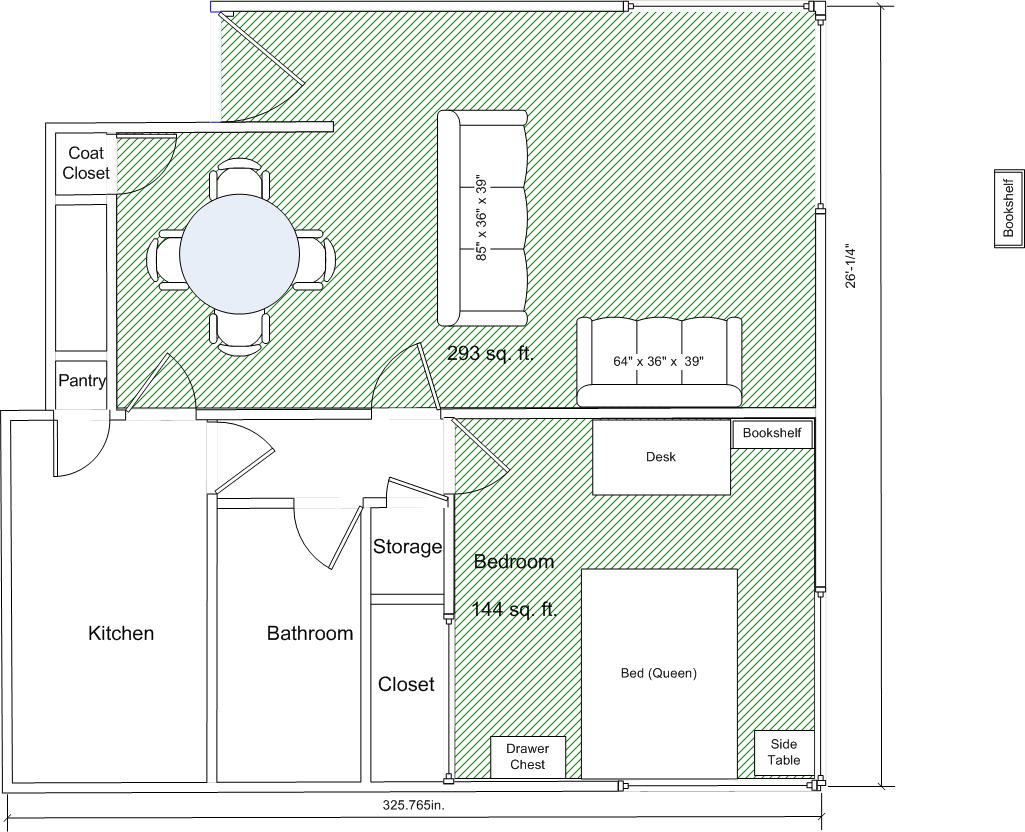This image features a detailed floor plan of an apartment. The layout begins at the entrance, leading to a series of clearly defined rooms. As you enter, you're greeted by a coat closet and a pantry, ideal for storage. Adjacent to this is a designated dining area, complete with a table accommodating four chairs.

The living room is spacious, depicted with a couch and a loveseat, leaving ample room for additional furniture or movement. The primary color palette of the apartment is predominantly white, accented by sections in the bedroom and great room that feature subtle light green stripes interspersed with black. 

Moving through the layout, you'll find a well-organized kitchen and a bathroom, both shown with storage options and a closet for added convenience. The bedroom is mapped out to be 144 square feet, with suggestions for arranging a bed, a bedside table, a chest of drawers, a desk, and a bookshelf, maximizing the functionality of the space.

The great room, measuring 293 square feet, is similarly detailed, with precise measurements for the couch and loveseat. Each furniture piece is meticulously measured to help visualize and plan the interior setup effectively. This floor plan is particularly useful for potential occupants, providing a comprehensive overview of the apartment's dimensions and the potential arrangement of furniture.